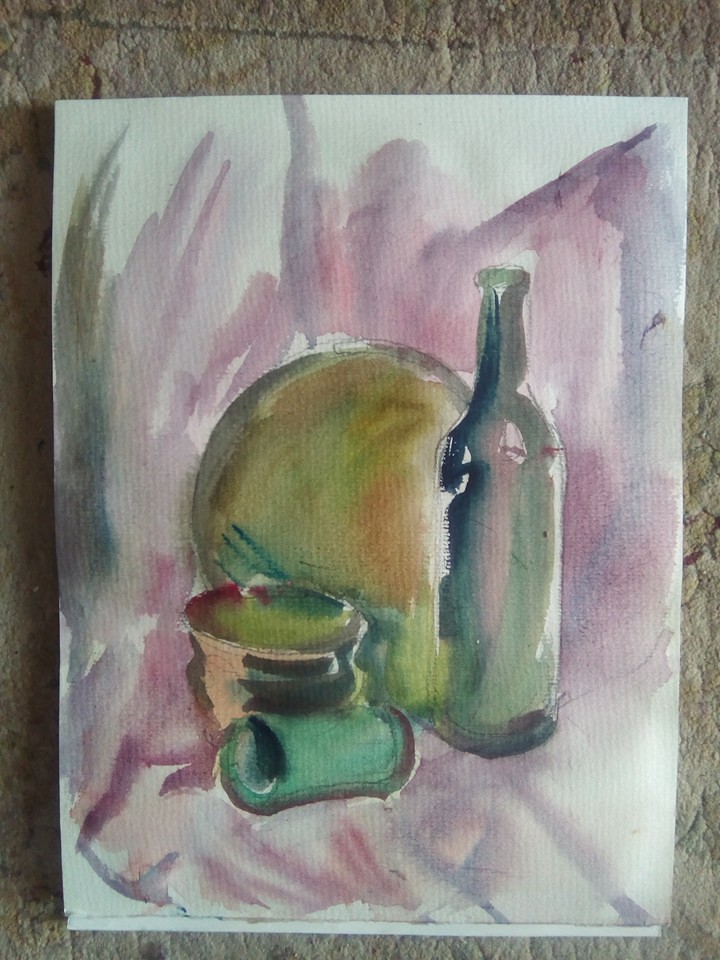This image showcases a delicate piece of watercolor artwork, seemingly painted on a sturdy piece of white cardboard. The artwork is presented in a close-up shot, either lying on a textured, stone-like surface or possibly displayed on a wall. At the center of the composition is an intricately detailed wine glass, which contains a round, greenish object. To the left and slightly in the foreground of the wine glass is a bowl, adding depth and perspective. In front of this bowl, on its side, is a green cup, drawing the viewer's eye into the layered arrangement of objects that exemplifies a still-life scene. The careful use of watercolors creates a sense of texture and light, highlighting the artist's skill in capturing the essence of everyday items in a refined and cohesive manner.